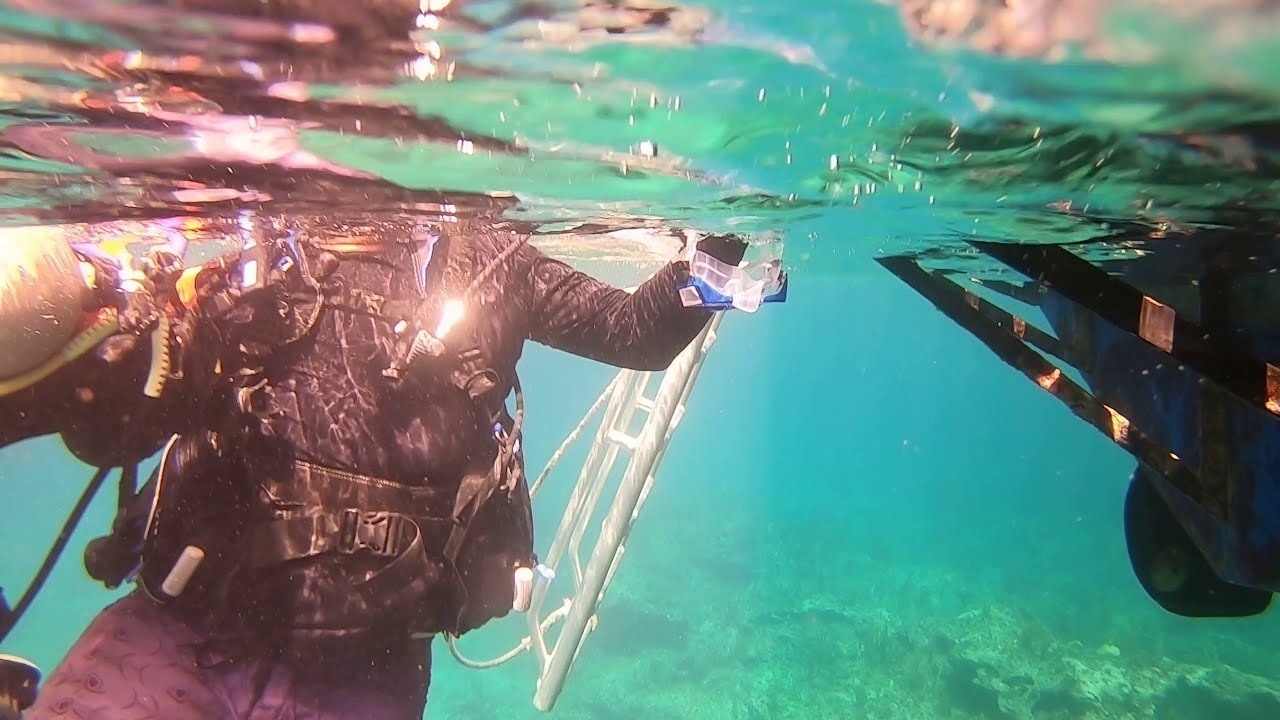This horizontal underwater photo captures a diver near the water's surface, where the top part of the image shows reflections from above and the water is a clear turquoise or greenish-blue hue. On the left side of the image, a person, whose head is not visible, is wearing a diving suit and a vest loaded with scuba gear, including heavy equipment resembling a tank or a welding contraption. The diver's left hand holds a clear and blue diving mask and they are gripping a small white ladder with a rope attached. On the right side of the image, partly submerged, there is a black and gold object, possibly the bottom part of a boat, along with two black straps connected to what resembles a navy blue bag or tool. The scene is illuminated by light coming through the water from above.